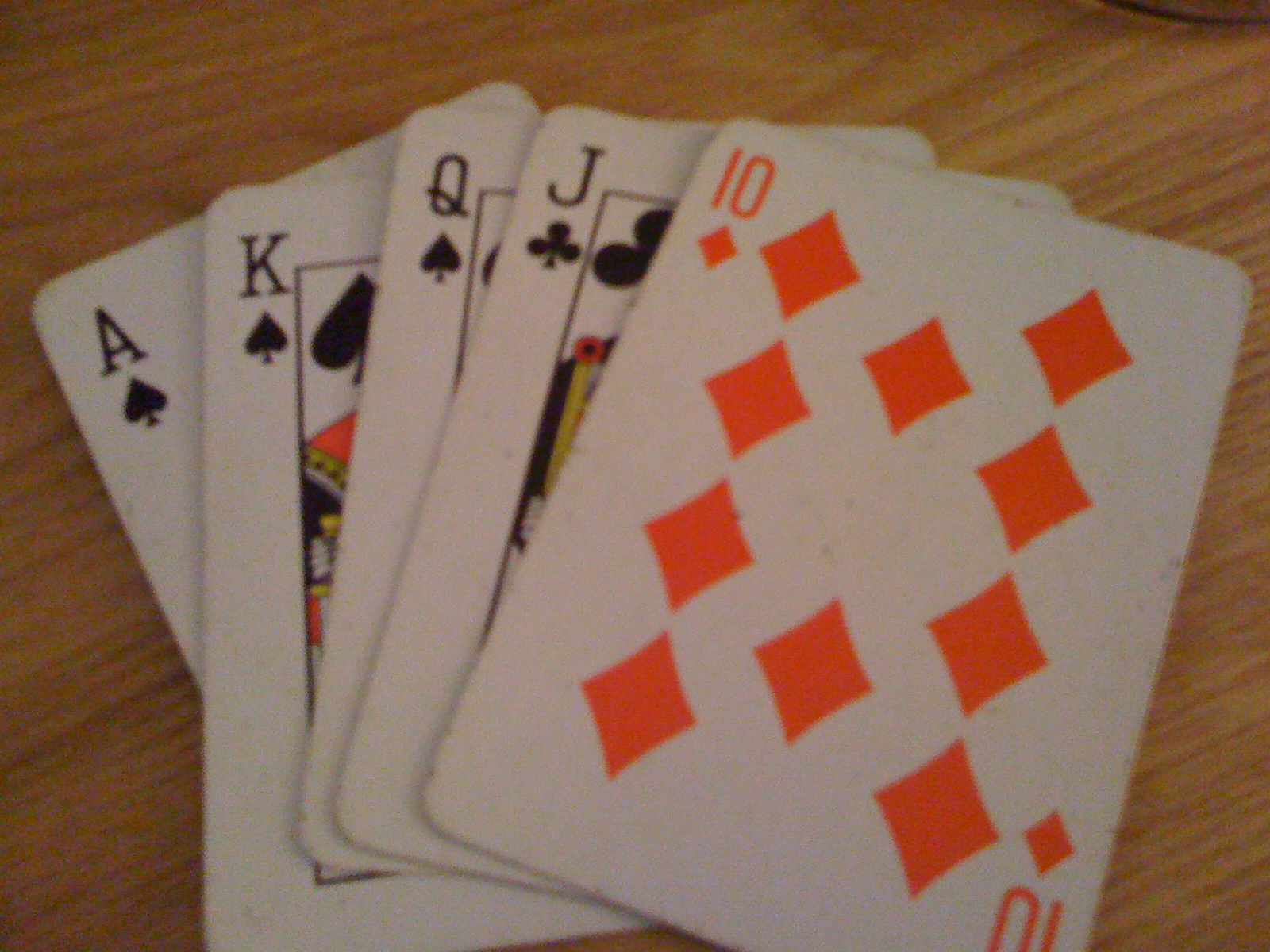The image is slightly wider than it is tall, approximately by 20%. The background seems to be a light wood surface, suggesting it might be a table, though this isn't certain. The wood grain features diagonally oriented striations, with one set pointing roughly towards seven o'clock and the other towards two o'clock. The wood appears seamless, with no visible board divisions.

In the center of the image, a hand of cards is prominently displayed, spanning almost completely from the left to the right edges and positioned about 10-15% down from the top. The bottom of the cards is cut off. The cards are fanned out as if being held in someone's hand, showing only the top left corners. The revealed cards form a straight, consisting of the ace of spades, king of spades, queen of spades, jack of clubs, and ten of diamonds. The cards also appear somewhat worn, with visible gray specks and slight markings suggesting frequent use.